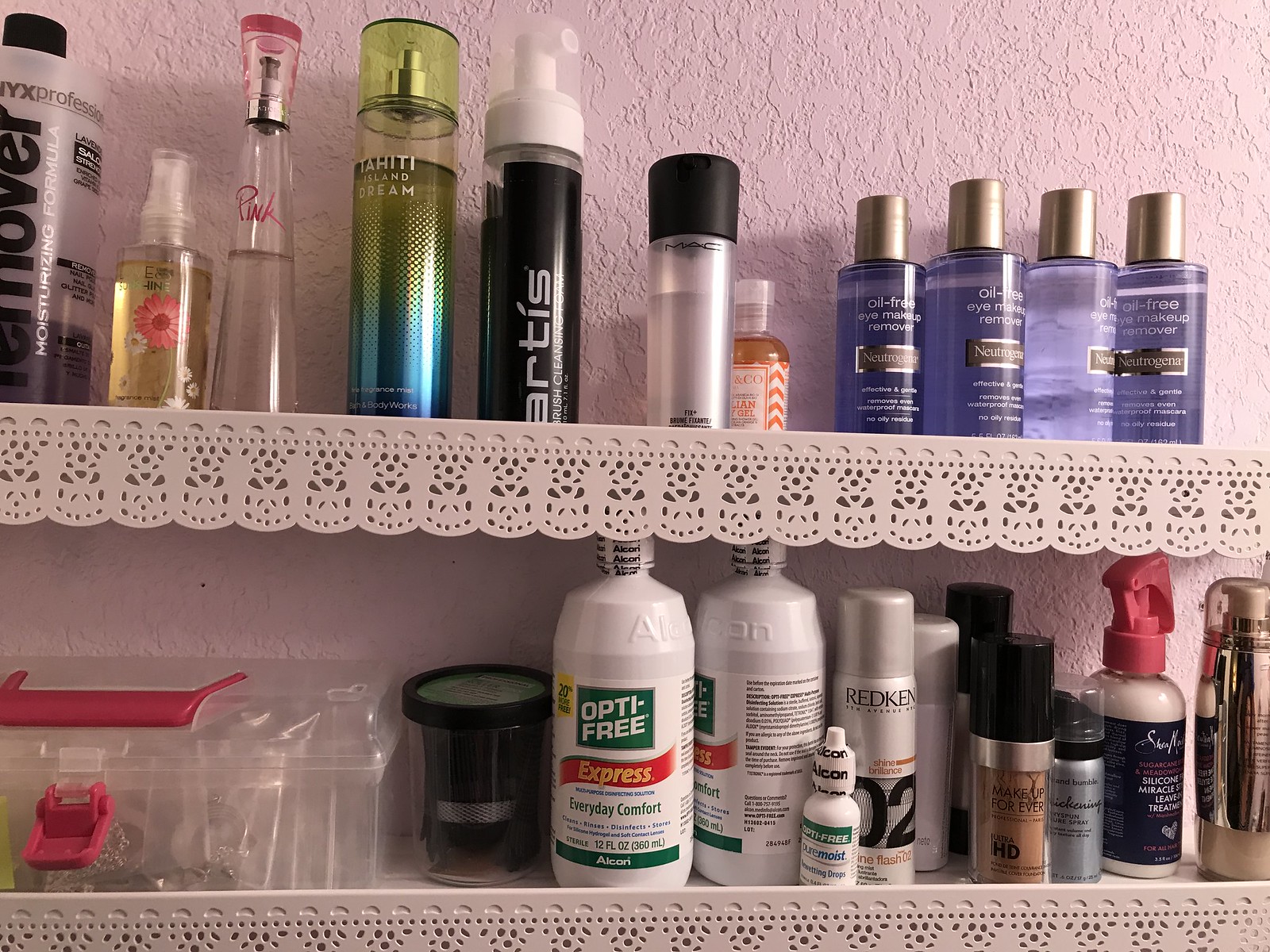A meticulously organized cabinet in a restroom, showcasing an assortment of personal care products. The cabinet features two white shelves against a light pink wall, adding a touch of elegance to the setting. On the bottom shelf, prominently positioned, is a bottle of Opti-Free Express Everyday Comfort Solution for contact lenses. Surrounding it are various skin creams and body sprays, their labels indistinct but hinting at a range of skincare essentials. The top shelf, equally well-organized, holds an array of items including a purple bottle with a gold screw cap, likely an oil-free makeup remover. Adjacent to this are multiple other beauty and skincare products typical of a woman’s personal care collection, suggesting makeup removers and skin conditioners. The overall scene is tidy and comprehensive, encapsulating the essentials of a well-appointed personal care nook.